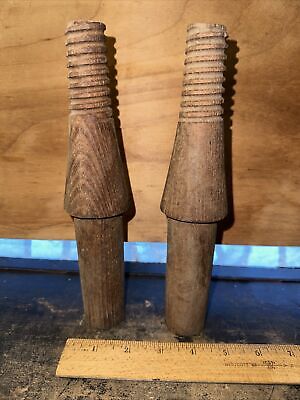This is a full-colored photo featuring two nearly identical wooden pegs displayed upright. The pegs, made of dark wood with visible grain texturing, have a cylindrical shape that is slightly irregular. The top half of each peg is intricately carved with deep, screw-like spirals, while the middle section flares out into a somewhat trapezoidal shape before narrowing back into a cylinder at the bottom. Behind the pegs, a light-colored wooden board and a faint, glowing blue stripe—likely from an adjacent window—are visible. The pegs are positioned on a black-painted tabletop, which appears distressed and worn to a lighter gray in the foreground. At the base of the wooden pegs lies a wooden ruler marked with inch increments, indicating that the pegs are just over an inch in diameter.